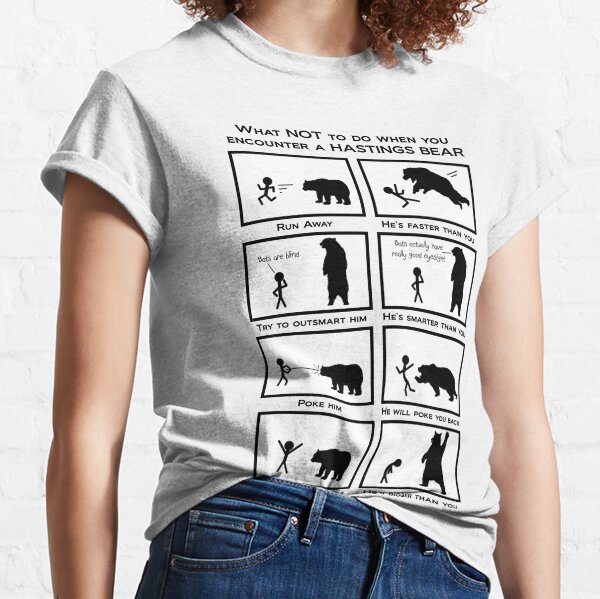This photograph captures a woman in a standing position, showcasing her upper body adorned in a light grey, short-sleeved t-shirt accompanied by blue jeans with no belt. Her long hair reaches down to her shoulders, though her face is not visible. The t-shirt features a black comic strip design offering humorous yet cautionary advice on how to behave when encountering a Hastings bear, outlined in a series of eight rectangles. The text at the top of the design reads, "What not to do when you encounter a Hastings bear." The comic illustrates various scenarios with accompanying advice such as, "Run away," showing a human silhouette fleeing from a bear, "He's faster than you," depicting a bear pouncing on a human, "Try to outsmart him," and "He's smarter than you," with respective visuals of a bear and human in different interactions. The final box warns, "He will poke you back," with an image of a human provoking a bear and the bear retaliating. The comical strip ends with a figure trying to scare the bear, emphasizing the humorous yet serious undertone of the comic. The background of the image is also light grey, complementing the t-shirt's color.